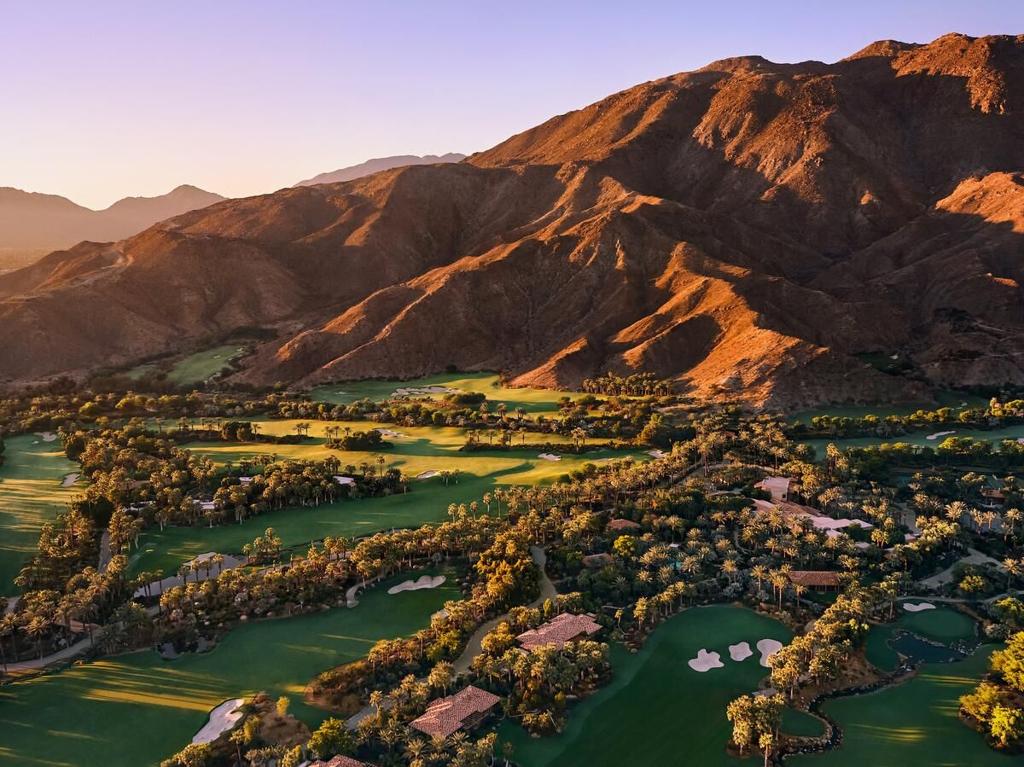An aerial or drone photograph captures an expansive golf course nestled in a picturesque mountainous area. The image highlights the vibrant green fairways and meticulously maintained greens, surrounded by dense clusters of trees that include various types of foliage, possibly palm trees. Numerous sand bunkers dot the course, with tree-lined fairways weaving between them. Embedded within the trees, scattered houses and structures are discernible, likely serving the needs of golfers and maintenance staff.

In the background, a striking red mountain range dominates the horizon, its undulating ridges illuminated by sunlight, perhaps indicating a sunset. Beyond this range, additional mountains fade into the distance, shrouded in a lighter, foggy hue. The sky above transitions from a whitish tint near the mountain peaks to a deeper blue as it stretches upward. The sunshine accentuates the greener fairways close to the mountains, creating a stark contrast with the darker, unlit grassy areas towards the bottom of the image. The overall composition draws the eye to the intricate design of the golf course, with tree-lined fairways radiating outward from a central point, blending harmoniously with the surrounding natural beauty.